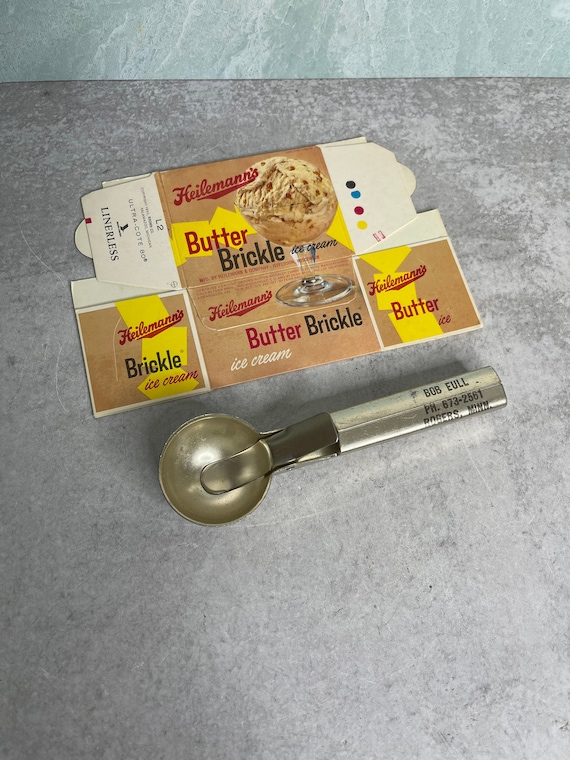The image is an overhead color photograph featuring a silver ice cream scoop and a flattened vintage ice cream carton, both set on a slate gray, possibly slightly greenish countertop. The ice cream scoop, displaying the name "Bob Eull" along with a phone number "673-2561" and the location "Rogers, Minnesota" on its handle, includes a lever mechanism designed to release the scooped contents. Above the scoop rests a flattened, brown pasteboard ice cream carton, with an old-fashioned design, likely from the mid-20th century. The brand "Hillman's" is prominently displayed in red cursive lettering, and the flavor "Butter Brickle Ice Cream" is clearly marked. The carton features an image of a large scoop of light brown ice cream with darker brown specks, showcased in a clear glass bowl. The packaging also has a background framed in hues of brown, yellow, and orange.